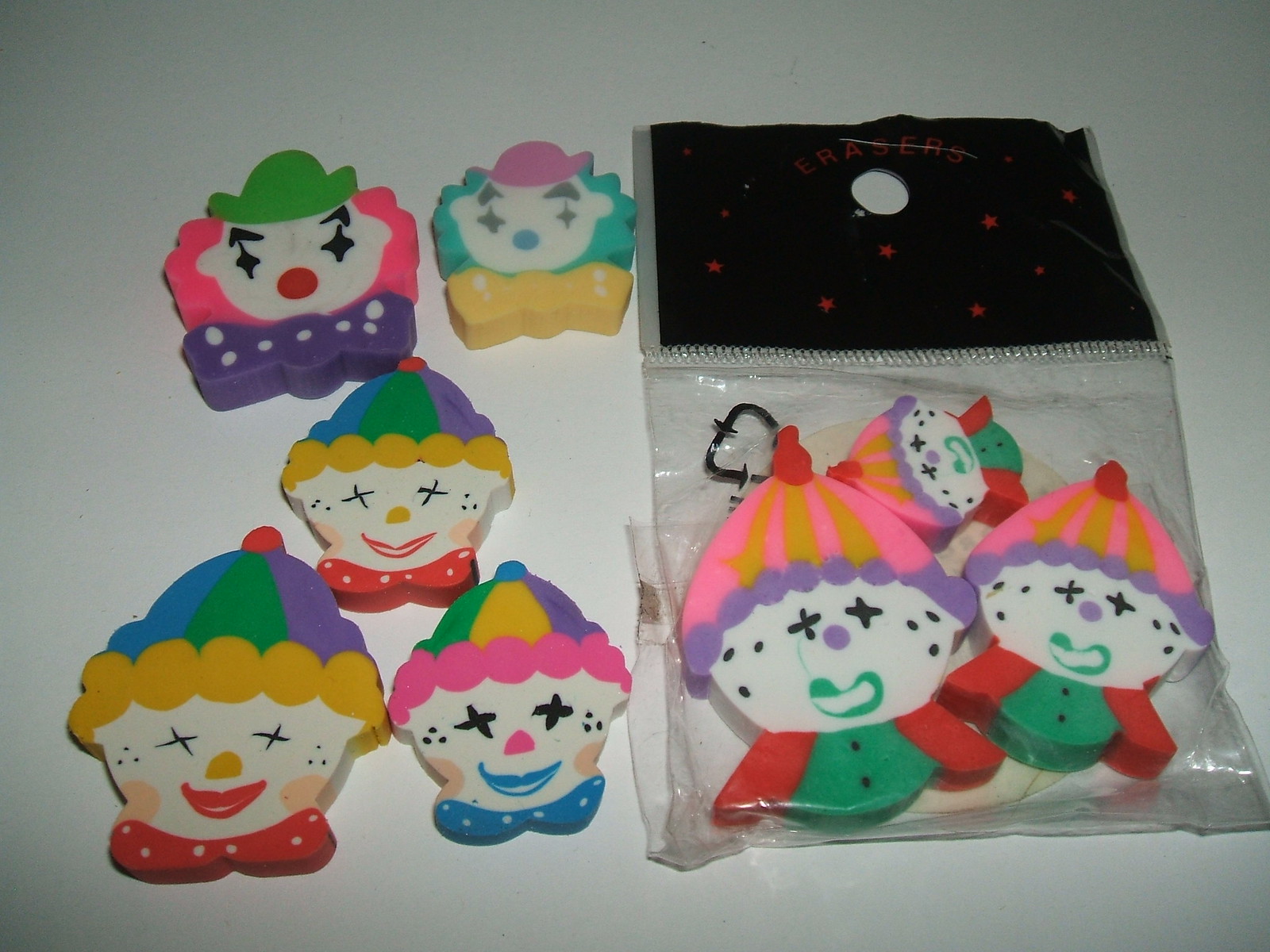The image depicts a detailed assortment of clown-themed pencil erasers. The erasers are vibrantly colored and shaped like clown heads, some also featuring upper bodies and arms. To the right, a see-through plastic package contains several clown erasers with eerie Xs for eyes, turquoise green mouths, and multicolored hats in shades of yellow, pink, and blue-green-purple. This package has a black top with red stars and is labeled "erasers." Outside the package, arranged to the left, are five standalone clown erasers. These clowns have variously colored hats in green, pink, purple, yellow, blue, and orange. Among these, the top two clown heads lack facial expressions, while the three below them are smiling. The overall scene is a vivid display of creepy yet colorful clown faces, with varieties distinguished by their distinctive hats, facial features, and packaging.